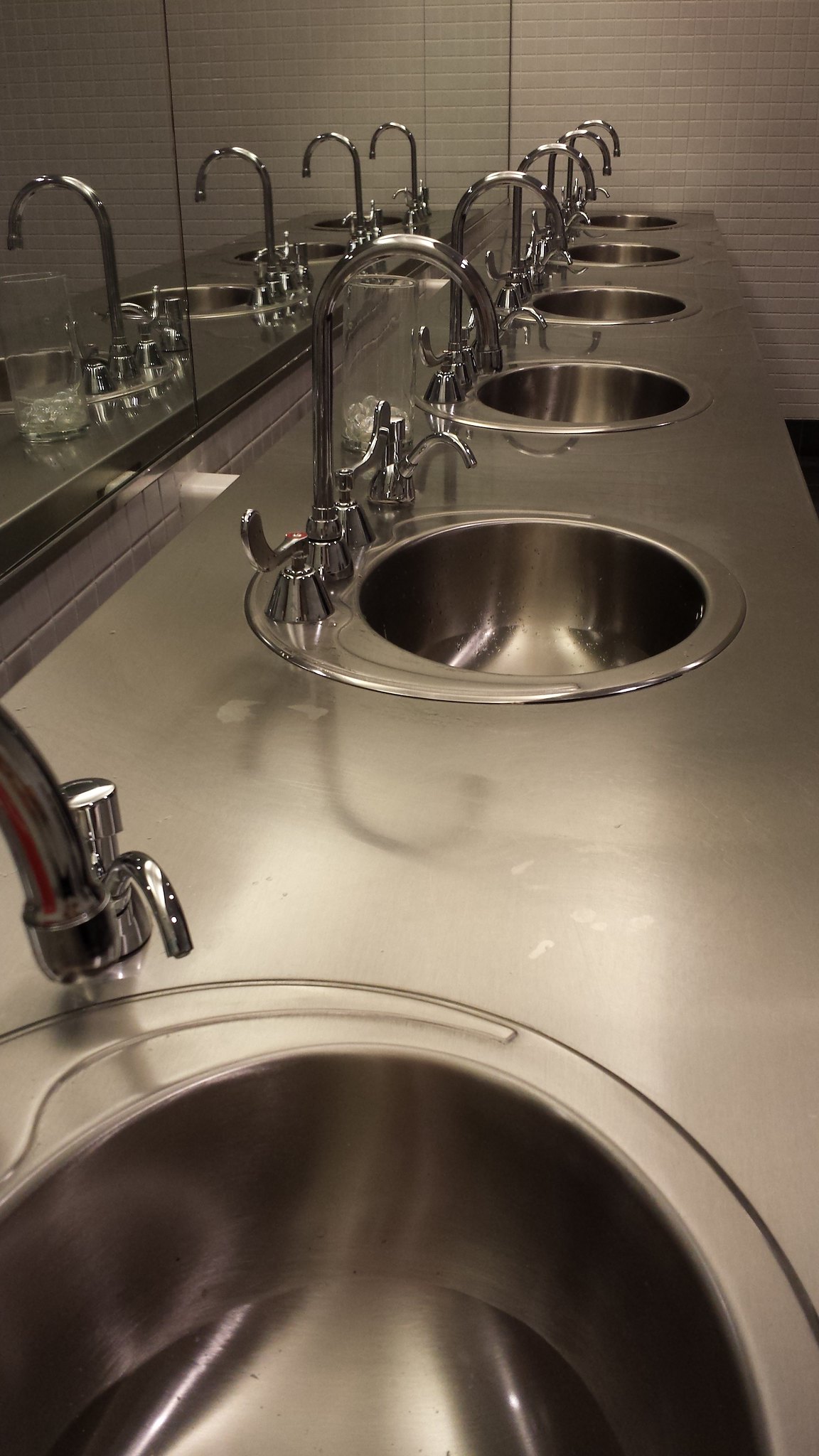The image depicts a row of six stainless steel sinks, each with dual-handled stainless steel faucets, aligned against a white tile wall. The sinks and countertops are crafted from a single piece of stainless steel, emphasizing a sleek, modern design. To the left of each sink is a stainless steel soap pump, maintaining the uniformity of the metal fixtures. A mirror, comprised of several panels, runs the entire length of the sink row, reflecting four of the faucets due to the angle of the photograph. The perspective of the image, taken vertically, showcases the sinks extending into the background, with the front sink appearing largest and each successive sink diminishing in size. Overhead lighting highlights the metal surfaces, creating a gleaming effect on the stainless steel. The setting suggests a high-traffic public restroom, possibly in a restaurant or shopping mall, designed to accommodate numerous users simultaneously.